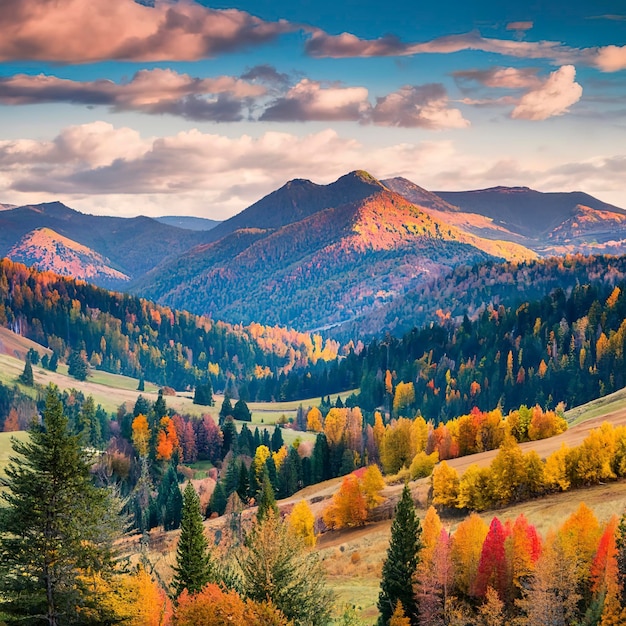This large square image, which could be an artistic print, computer-generated, or a photograph, captures a breathtaking fall scene in a mountainous countryside. The landscape is painted with rich autumn colors and detailed layers of natural elements. 

The foreground features a variety of trees, including evergreens and hardwoods, in vibrant shades of red, yellow, green, and orange. On the left side, a large green tree stands out among yellowish bushes and other green trees, while the right side showcases a colorful mix of green, yellow, pink, and red small trees.

As the scenery recedes into the midground, the landscape transitions into hilly terrains with dense clusters of green pine trees interspersed with orange-tipped conifers. The hills on the right rise steeply, dotted with yellow, pink, and orange trees, while those on the left descend into a valley filled with green vegetation. The middle ground features open grassland hills, rising and falling gently, leading the eye towards dense wooded areas of orange and green trees in the distance.

The background is dominated by mountain ranges with brownish outlines and green patches of trees at their sides. Above the mountains, the sky is a canvas of ever-changing clouds, with three distinct horizontal layers in hues of white, gray, and even some brown, interspersed with blue sky. The light blue transitions into a lighter shade towards the horizon, adding depth to the expansive view.

The entire scene is bathed in sunlight, highlighting the vivid colors of the changing foliage and casting a warm, enchanting glow over the picturesque landscape. The contrasting palette of the trees and the harmonious blend of the mountainous and hilly contours create a mesmerizing, almost surreal autumn vista.